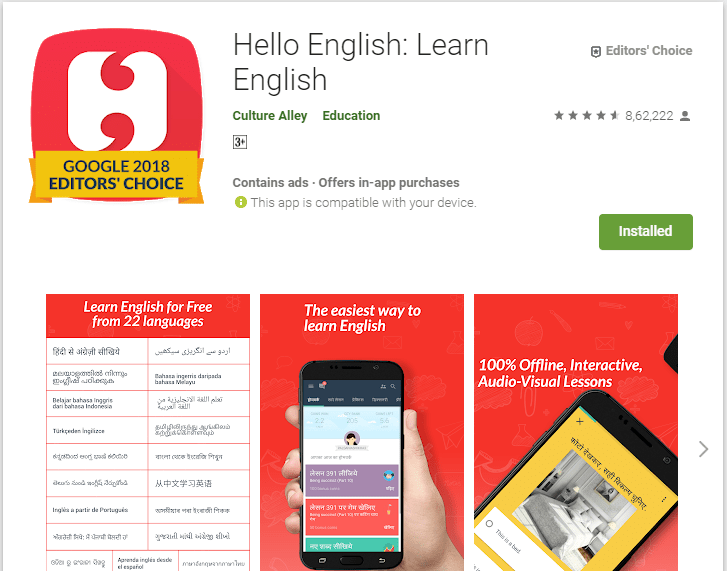At the top left of the image, there's an icon with a red background resembling the letter "H" or two apostrophes, one inverted above the other. Below this icon, a yellow ribbon displays the text "Google 2018 Editor's Choice." To the right, there is the title "Hello English: Learn English" followed by "Culture Alley Education" for ages "3+." Further down, it mentions that the app contains ads and offers in-app purchases. Additionally, it states that the app is "compatible with your device" and is an "Editor's Choice" selection, with a rating of approximately four and a half stars from 862,222 reviews. A green bar indicating "Installed" is visible, implying the app is already on the user's device.

Below this section, on the left, there's a statement that reads "Learn English for Free in 22 Languages," followed by a box displaying two rows of various languages written in different characters. On the right, a smartphone is depicted in someone's hand, with the text at the top declaring "The Easiest Way to Learn English." Further down, another smartphone is shown resting on a red surface, with a caption that reads "100% Offline Interactive Audio-Visual Lessons."